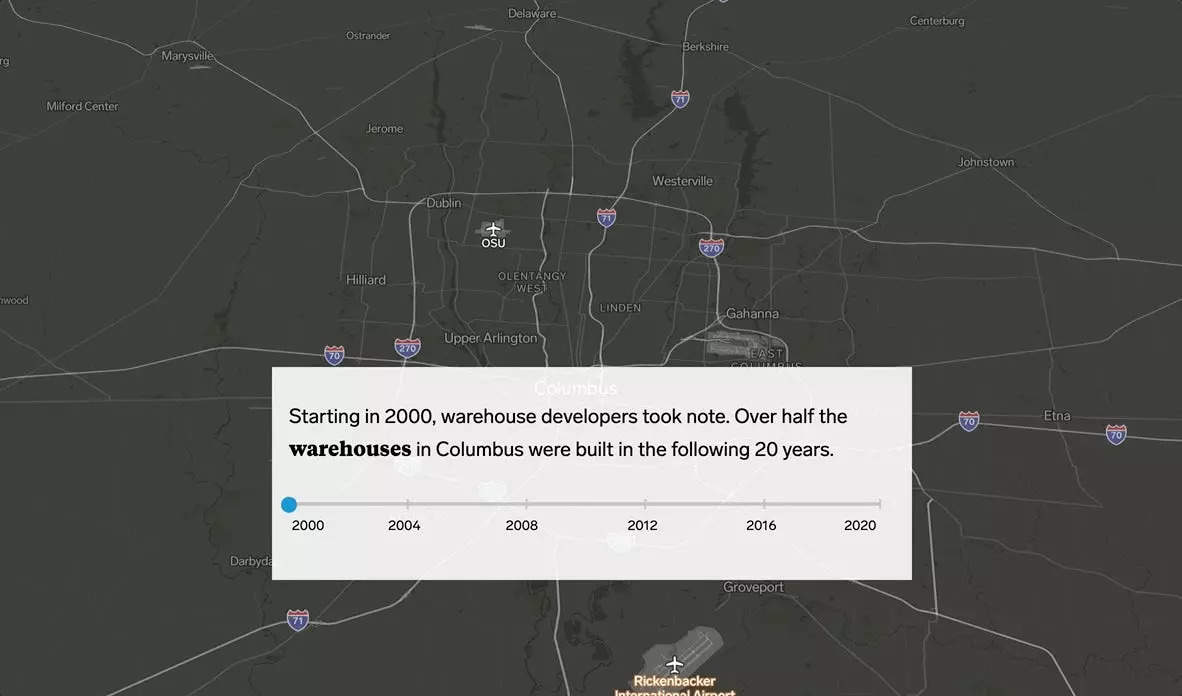Screenshot of a website featuring a grayish backdrop, depicting a map outlined with multiple white lines to signify geographical boundaries. Centered slightly towards the bottom, there is a prominent white pop-up box with text in black: "Starting in 2000, warehouse developers took note. Over half of the warehouses in Columbus were built in the following 20 years." Below this statement, the word "warehouses" appears in bold.

Inside the white box, a long gray progress bar stretches horizontally, topped with a blue draggable circle positioned on the left. This interactive element allows users to adjust the date range between 2000 and 2020, demarcated by dates 2000, 2004, 2008, 2012, 2016, and 2020, each written in black.

Scattered across the gray map backdrop are small shield symbols, colored red on top and blue on the bottom, representing the United States interstate system. At the bottom center of the image, an airplane icon is placed above the text "Rickenbacker" in white, followed by "International Airport."